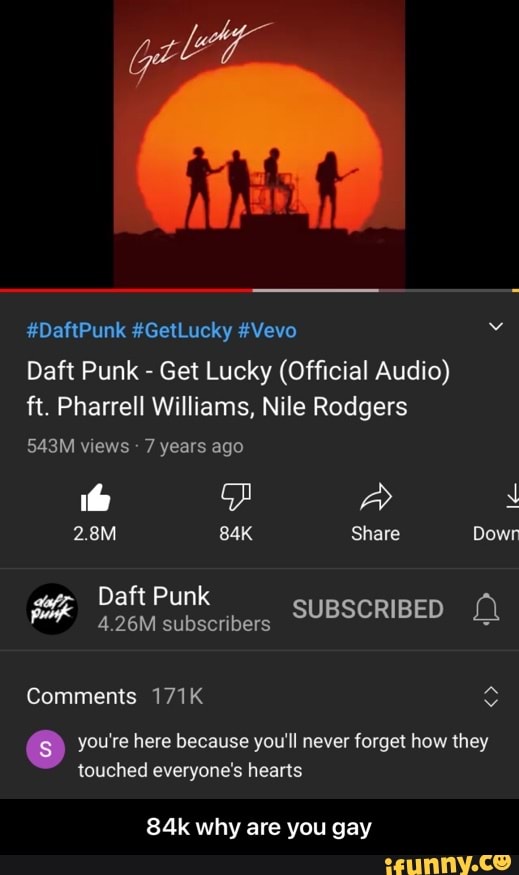A detailed snapshot of a social media page features a vibrant image of a band performing against a captivating sunset backdrop. To the left of the image, there is a prominent text mentioning "Get Lucky." Surrounding this visual are various descriptive tags including "Daft Punk," "Get Lucky," "Bevo," and more specifically, "Daft Punk - Get Lucky (Official Audio) featuring Pharrell Williams and Nile Rodgers." The audio itself has garnered substantial attention, having been viewed 543 million times over the past seven years, with 2.8 million likes and 4.26 million subscribers to Daft Punk's channel. Additionally, there are a staggering 171,000 comments, many of which express sentiments such as "You're here because you'll never forget how they touched everyone's hearts." A noticeable black banner at the bottom of the screen reads "84K, Why Are You Gay?" Lastly, in the bottom right-hand corner, the recognizable yellow "ifunny.co" logo is displayed.